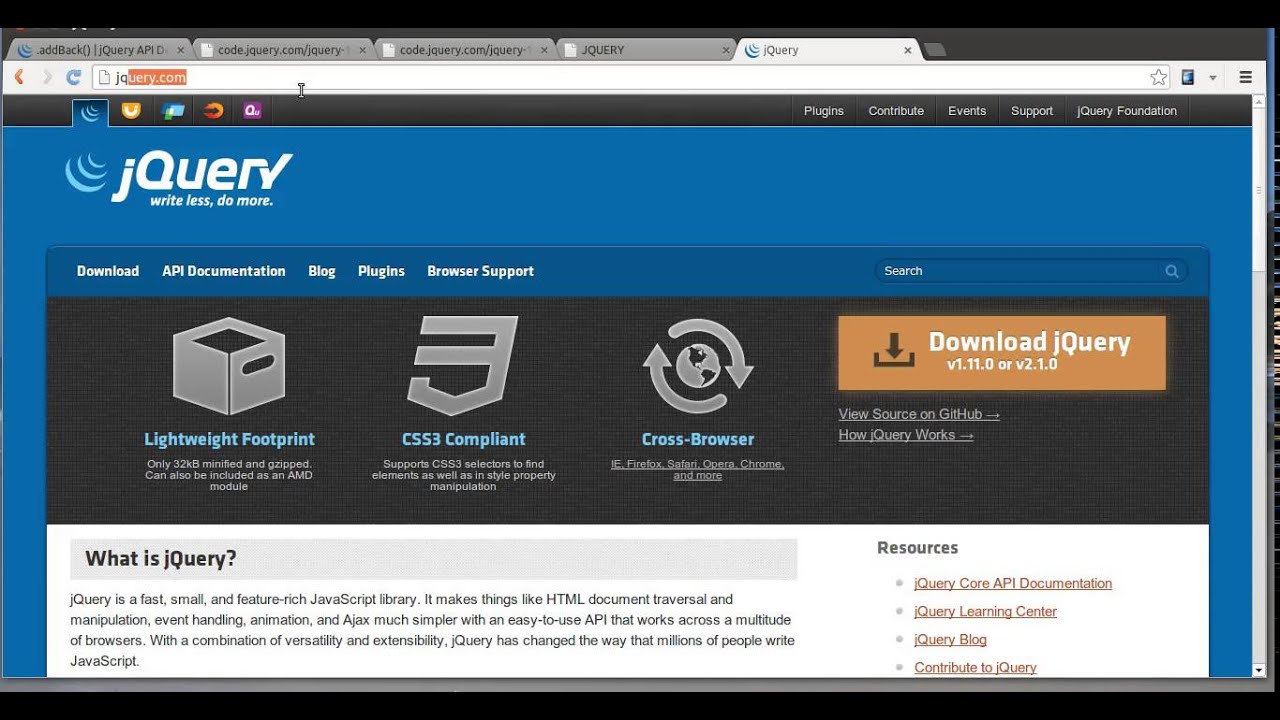In the web search image, there are four adjacent tabs visible alongside the main search. The displayed content prominently highlights the slogan "Write Less, Do More" associated with jQuery. The accompanying options include Plugins, Contribute, Events, Support, and the jQuery Foundation. Further highlighted sections include "Download," "API Documentations," "Blog," "Plugins," "Browser Support," and a search function. 

The jQuery library is noted for its lightweight footprint, being only 32 kilobytes when minified and gzipped, applicable as an AMD module, and compliant with CC3. It supports CSS3 selectors and various runtime environments, featuring overall style properties and cross-browser compatibility with Firefox, Safari, Opera, Chrome, and others. Users are prompted to download jQuery versions v1.11.0 or v2.1.0 and view the source on GitHub. Additional resources explain "How jQuery Works" and answer "What is jQuery?"